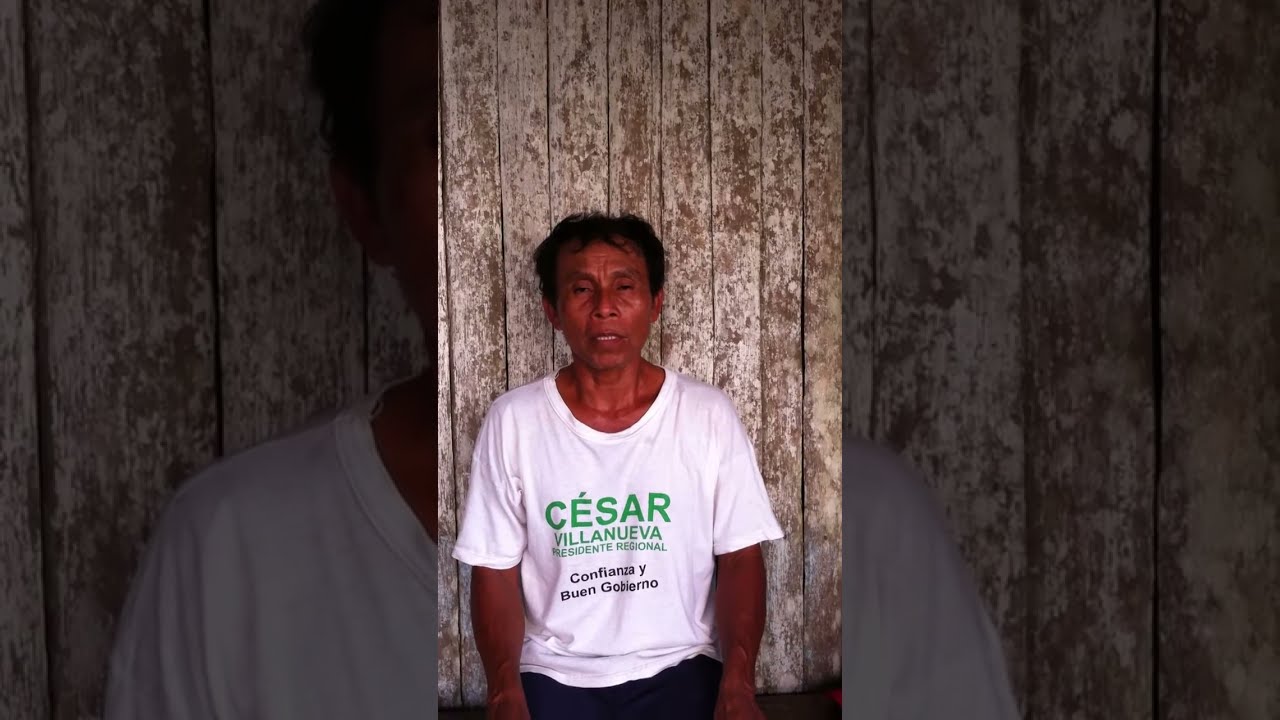A dark-skinned man with short black hair is leaning against a weathered wooden wall that appears to have once been white but now displays numerous brown spots. He has a neutral expression with possibly closed eyes and is wearing a white t-shirt with green and black lettering. The shirt reads "César Villanueva, Presidente Regional, Confianza y Buen Gobierno." His arms are down by his side, and his hands are not visible, possibly in his pockets. The image captures him from the waist up against the backdrop of the damaged, discolored fence-like wall.